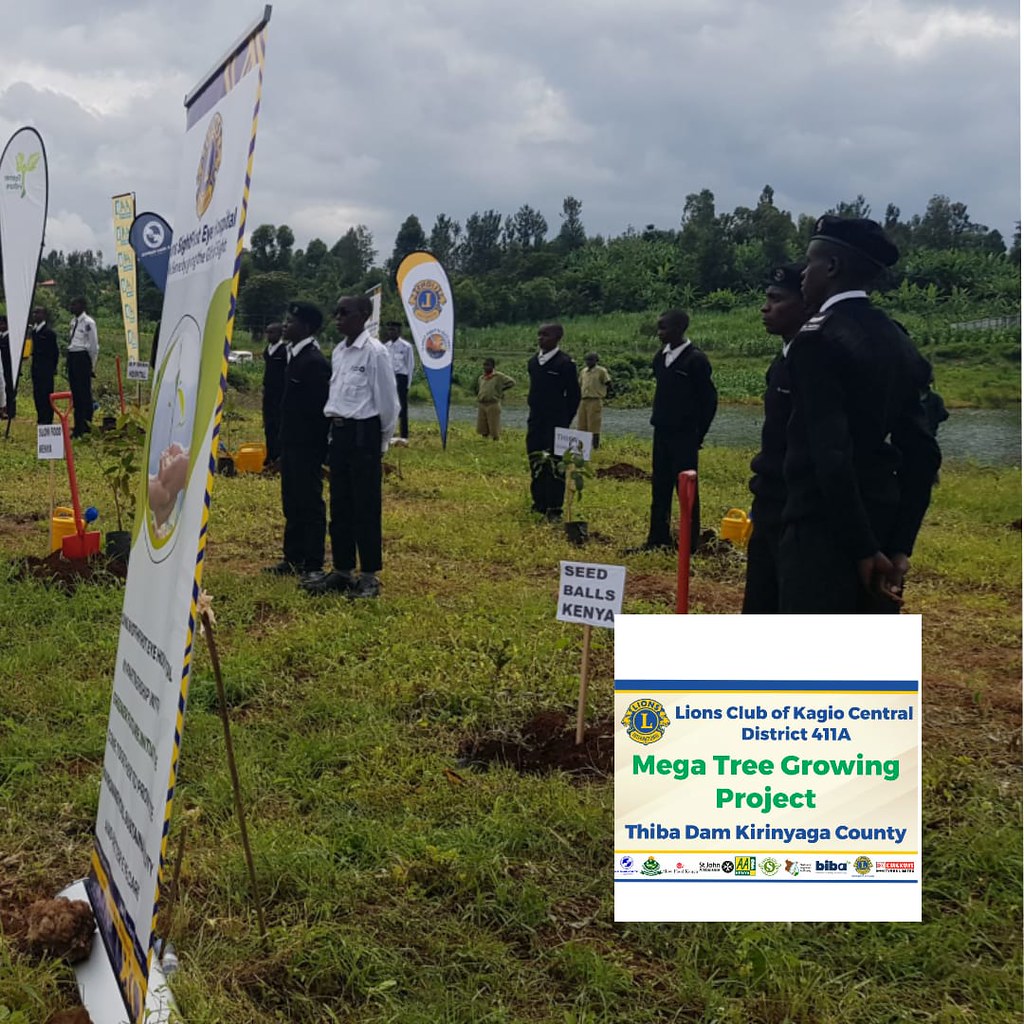This photograph captures a ceremonial tree planting event held in a grassy field, presumably in Kenya, as indicated by the signs and attendees' attire. The central focus is a large sign that reads "Lions Club of Coggio Central District 411A Mega Tree Growing Project, Theba Dam, Coringa County," accompanied by multiple smaller signs advertising the same project, and another sign that says "Seed Balls, Kenya." 

The participants, a diverse group of individuals primarily consisting of African men and possibly women, are dressed in varying uniforms suggesting a mix of military personnel and junior cadets. The military individuals are identifiable by their khaki uniforms and black berets, while others, likely cadets, wear black sweaters or black pants paired with white dress shirts and black berets. Some children are seen in neat formal uniforms, hinting at their participation in a training or educational program.

The participants are mainly standing in pairs next to newly planted trees, and they all seem to be gazing off into the distance, enhancing the sense of ceremony. The background features a marsh pond, adding an element of natural beauty to the scene. The presence of the Lions Club flag and the prominent lion symbol emphasize the organizational support behind this environmentally focused event.